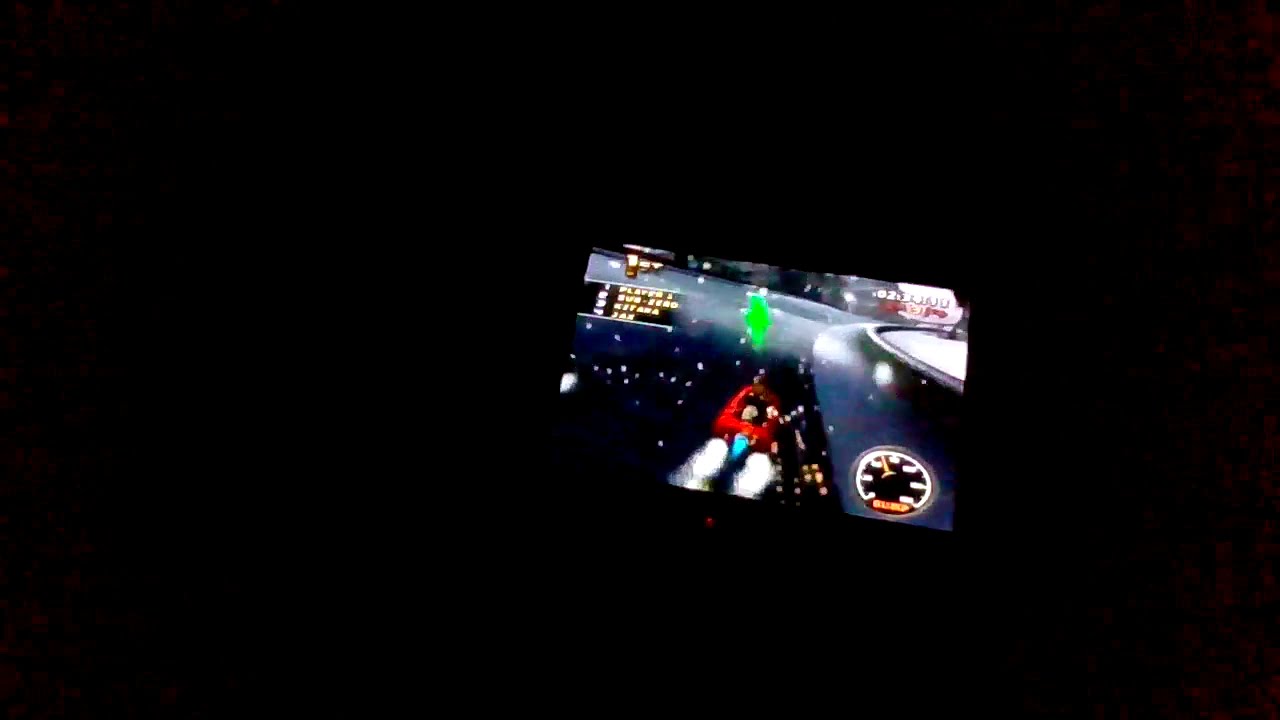Against a very large black background, there is a square photo that is tilted slightly to the right. The photo seems to be a screenshot from a video game, possibly a racing game. In the bottom right corner of the image is a round gauge, resembling a speedometer, with a yellow marker pointing slightly up and to the left. The gauge displays seven sets of white numbers, with the word "bump" written in bright orange underneath it. The gauge's background is black.

In the upper left corner of the photo, there is a square with yellow lettering that is difficult to read, containing four lines of text. The first line mentions something about a player, the second says "sub-zero," and the last line includes the word "jar." Adjacent to these lines, white numbers are present. 

Centrally located in the image, there is a noticeable green spot that looks like a splatter of paint. Below this green spot appears to be a space or racing vehicle, characterized by jet propulsion and smoke trailing from two exhaust pipes, with a background filled with stars, suggesting a space race. The vehicle itself seems to be red. In the upper right corner, some white numbers are barely legible, including "0234."

Overall, despite the slight blurriness and small size of the screen capture, the image captures the essence of an in-game moment with an analog meter and a futuristic racing vehicle amidst a starry backdrop.